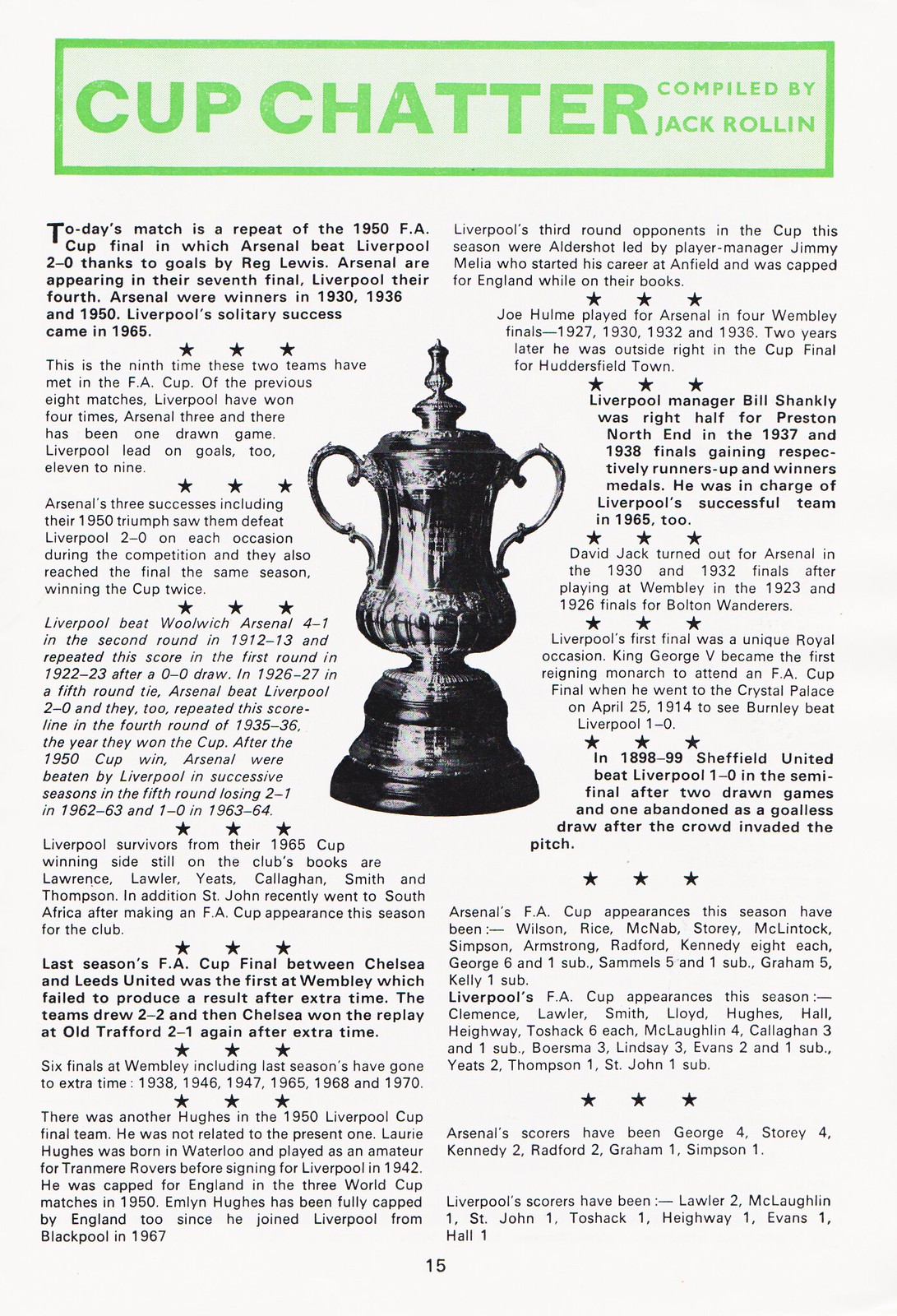This image is a detailed poster or single-sheet piece with the title "Cup Chatter" compiled by Jack Rollin, prominently displayed at the top in green letters with a slight green background. The poster is dedicated to various historical facts and trivia about Arsenal Football Club's FA Cup appearances and notable matches. The content is organized into multiple short paragraphs, each separated by three black stars, containing snippets of information.

In the top left corner, the text reads: "Today's match is a repeat of the 1950 FA Cup Final in which Arsenal beat Liverpool 2-0, thanks to goals by Reg Lewis." It also mentions Arsenal's previous title wins in 1930, 1936, and 1950, and Liverpool's solitary success in 1965. Another highlighted paragraph states: "This is the ninth time these teams have met in the FA Cup. Of the previous eight matches, Liverpool have won four times, Arsenal three, and one match ended in a draw." Additional trivia includes the fact that six finals at Wembley have gone to extra time, citing specific years such as 1938, 1946, 1947, 1965, 1968, and 1970.

The poster is text-heavy and split into two columns housing multiple paragraphs. Central to these columns is an image of what appears to be the FA Cup trophy, enhancing the historical and celebratory tone of the piece. This layout suggests it might be a page from a magazine or newspaper, compiling rich statistical data and anecdotes about Arsenal's FA Cup history.